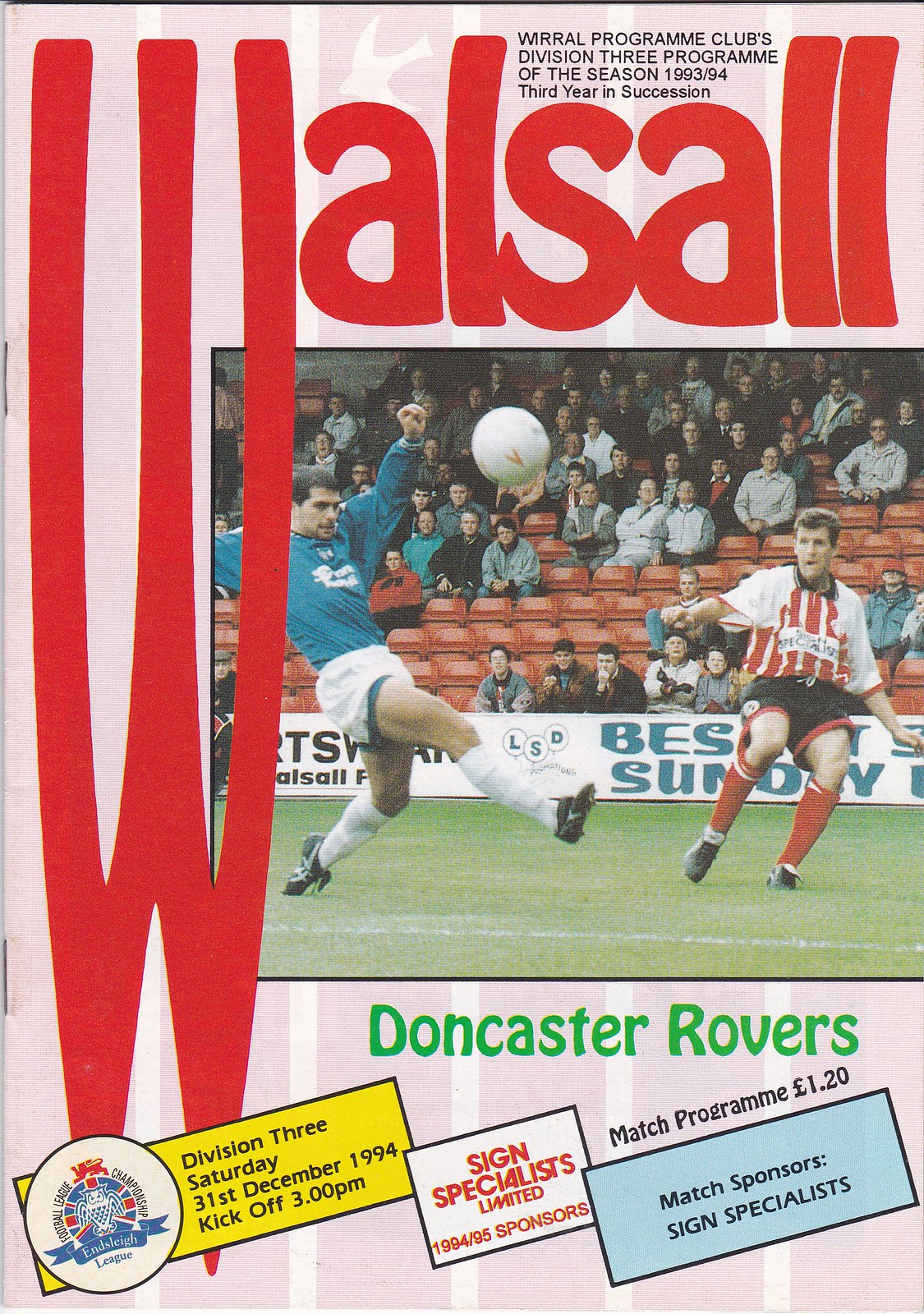This vertically aligned rectangular image is the cover of a Doncaster Rovers program booklet, held together by two staples along the left spine. Dominating the left side is an enormous red "W," stretching from top to bottom. At the top, in smaller red letters, is the rest of the word "WALSALL." Above this, in small black print, the cover reads: "WRRAL Program Clubs, Division III Program of the Season, 1993/94, third year in succession."

Central to the cover is a square, color photograph depicting a lively soccer scene. A player wearing a blue long-sleeve shirt and white shorts is captured mid-action, kicking a white soccer ball into the air. Opposing him is a player in a white jersey with red stripes, black shorts, and red socks, seemingly attempting to block the move. The background reveals an audience in orange seats, with some noticeable empty spots, hinting at a less-than-full stadium.

Beneath the photograph, green text boldly states "Doncaster Rovers." At the very bottom, three diagonally placed rectangles act as sponsor logos. The left rectangle mentions "Division III, Saturday, 31st December 1994, kickoff 3 PM." The middle rectangle highlights "Sign Specialists Limited Sponsors," and the rightmost rectangle designates "Match Sponsors, Sign Specialists." Additionally, the cover notes a price of "Match Program £1.20."